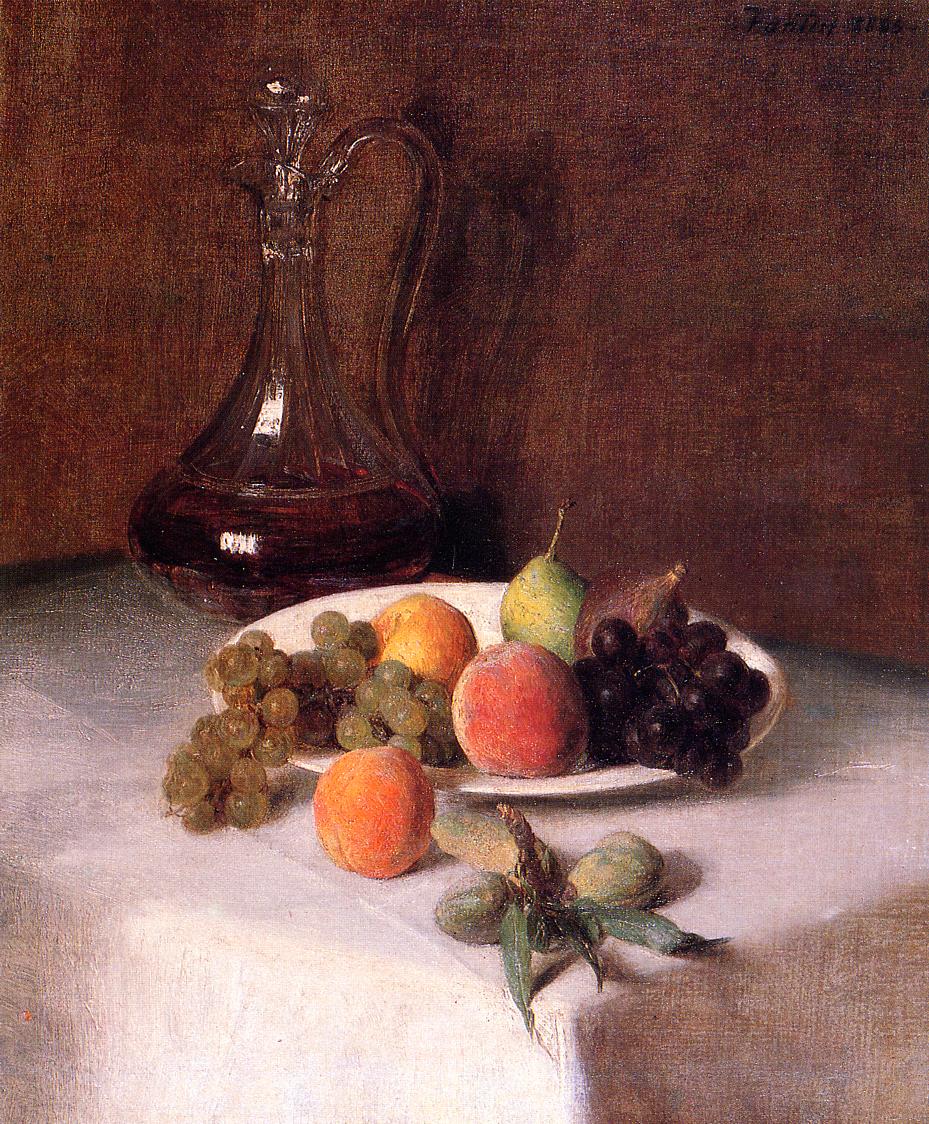This still life painting, likely an oil painting, is a highly detailed and photorealistic portrayal of a table decorated with a variety of fruits. The table is covered with a pristine white tablecloth, and the background comprises a muted brown wall, casting soft shadows that suggest a warm, ambient light source. At the center of this round or square table lies a white plate, meticulously arranged with green grapes on the left, black (or purple) grapes on the right, a pear, a couple of peaches—one of which rests directly on the table—and a fig or two near the front edge. 

Flanking the plate is an ornate glass pitcher with a gracefully curved handle, containing a dark liquid that might be wine or a similar beverage, showing a rich maroon hue. The liquid settles at the bottom, possibly due to the piece’s worn texture suggestive of an older painting. Near the edge of the table and accompanied by the cluster of fruits, there appears to be a piece of fruit with leaves attached. The backdrop also reveals the shadows cast by the pitcher, enhancing the depth and realism of the composition. A barely legible signature is discernible in the upper right corner, hinting at the artist behind this striking and timeless piece.